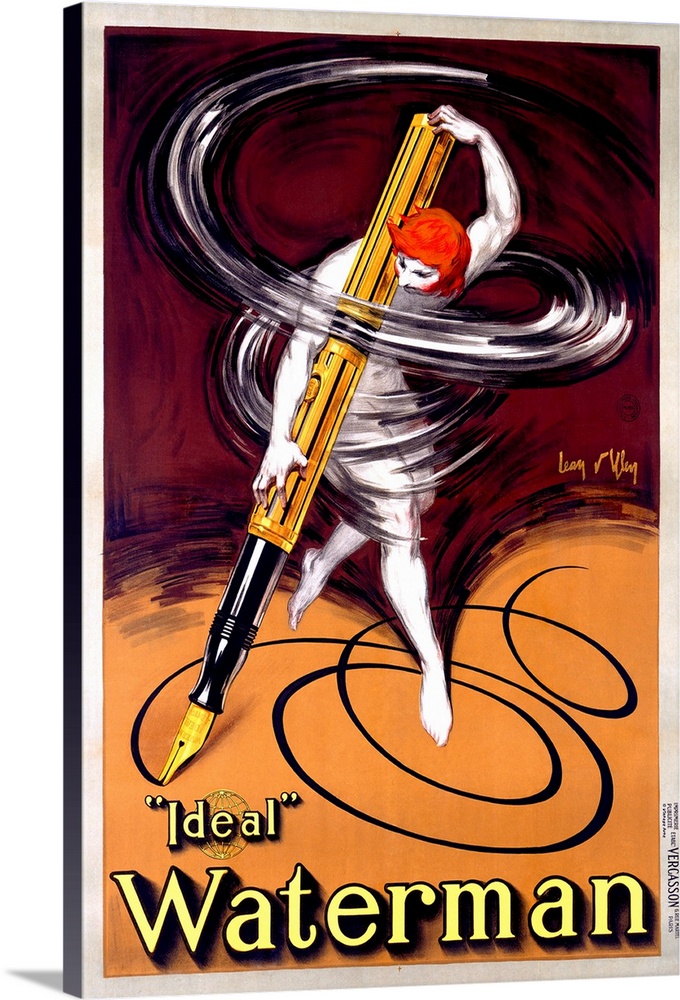This artwork, presumably a framed print or postcard, depicts a striking figure set against a rich maroon backdrop that transitions to a terracotta or clay brown hue towards the lower part of the image. The central figure, resembling a white marble statue with red, Jesus-style hair, leans forward holding an exaggeratedly large yellow pen. The pen, featuring a contrasting black cap, makes contact with the ground, leaving swirling marks that spiral around and behind the figure, giving an impression of movement. The background showcases a blend of dark orange and magenta textures, painted to mimic swirling motions. Positioned at the bottom of the image, text reads “Ideal Waterman” in yellow with a black shadow, while a signature of the artist, “Ver Cason,” appears within the artwork. The entire piece is bordered by a silver frame, set against a white background, with decorative edging along the lower right edge.